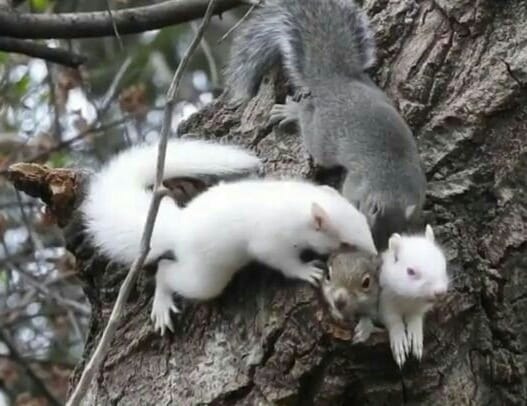In this detailed photograph, four squirrels are engaging with a textured, thickly-barked tree trunk in a forest setting. The squirrels consist of two grey squirrels and two white squirrels, the latter being albino and boasting strikingly bright white fur along with bushy white tails, feet, and hands. On the left side of the tree, one albino squirrel clings to the bark and seems to interact closely with a grey squirrel positioned nearby. Just below them, a small burrow is visible within the trunk, from which another pair of squirrels, one grey and one white, are peeking out. The grey squirrel outside appears to be attempting to join the duo nestled inside the hollow. The background shows a blurred mix of green foliage and brown tree branches, enhancing the natural forest atmosphere surrounding this lively squirrel interaction.